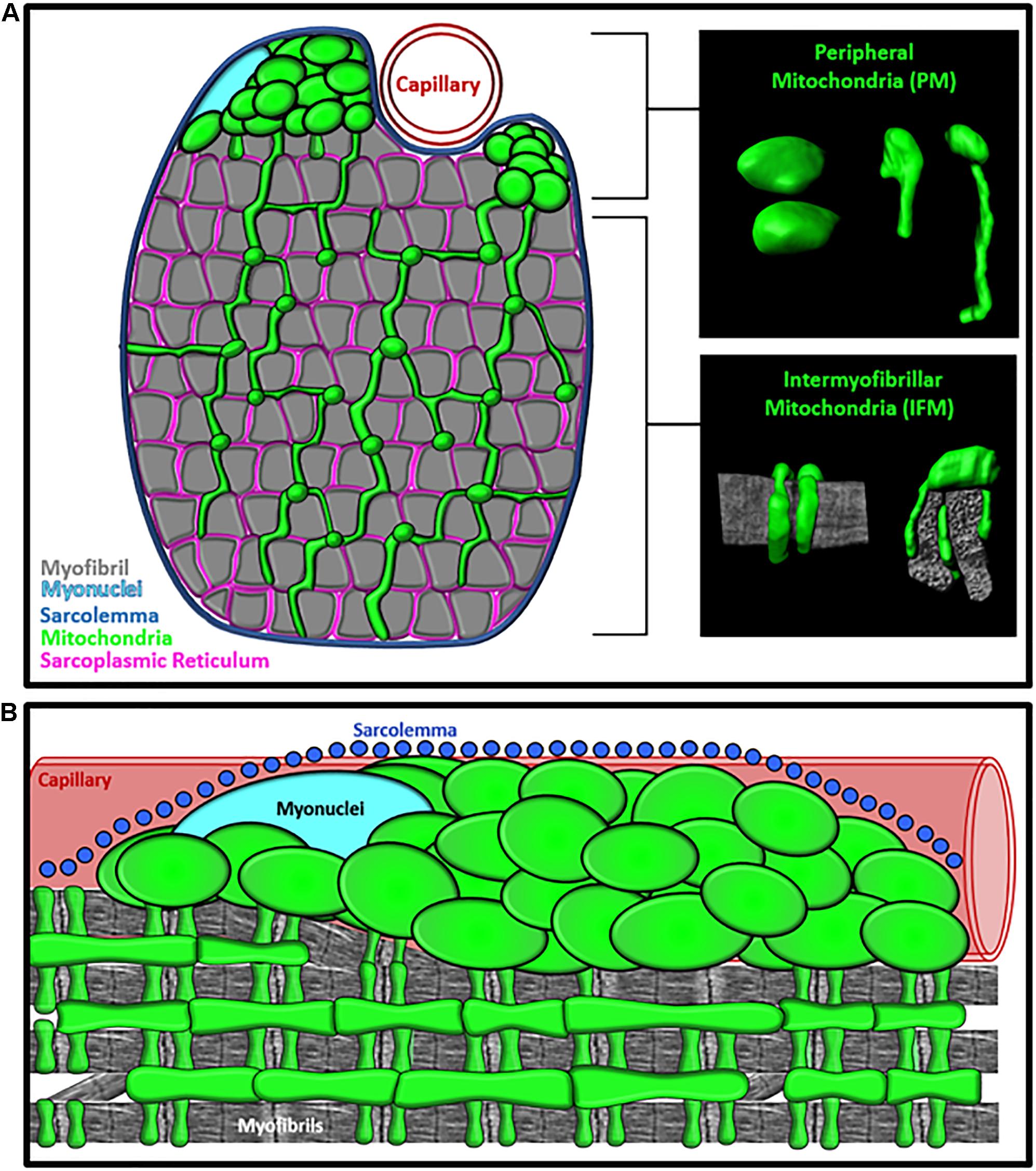This is a detailed, colorful drawing illustrating the structure of a capillary and associated cellular components within two distinct rectangular sections. The top section prominently features a large gray capillary with small green, pea-like myofibrils flowing through it. Labelled areas include "capillary myofibril" and "peripheral mitochondria," depicted as small, green, pea-like structures, as well as "intermyofibrillar mitochondria," illustrated as elongated green shapes. The background here is predominantly purple, while black squares highlight key terms. The lower section showcases the cell's intricate details, such as the "sarcolemma," which has a thatched, woven appearance and vibrant green, egg-shaped structures sitting atop it. The term "myonuclei" is also highlighted in this area. The overall image effectively uses a mix of colors, including light blue and pink backgrounds, to differentiate and emphasize various cellular components.